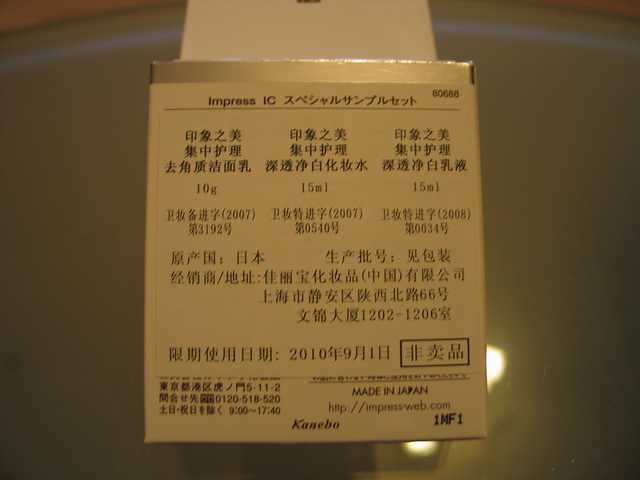The image depicts a white, square box prominently featuring Japanese kanji characters. The top of the box displays the text "Impress IC," while the bottom reads "Made in Japan, Impressweb.com, Kanebo, K-A-N-E-B-O, I-M-F-1," followed by a code. The box appears to be suspended or hanging, though the exact mechanism is unclear. In the background, lights are reflected on the surface of whatever is supporting the box, hinting at a possibly dark or glossy setting. This setting might be a museum or public display area, indicated by the dark brown background resembling a podium or stand typically used for exhibits. The label is written almost entirely in Japanese, with three groupings of kanji characters followed by descriptions. The foreground prominently features this label, positioned clearly for viewers to read.